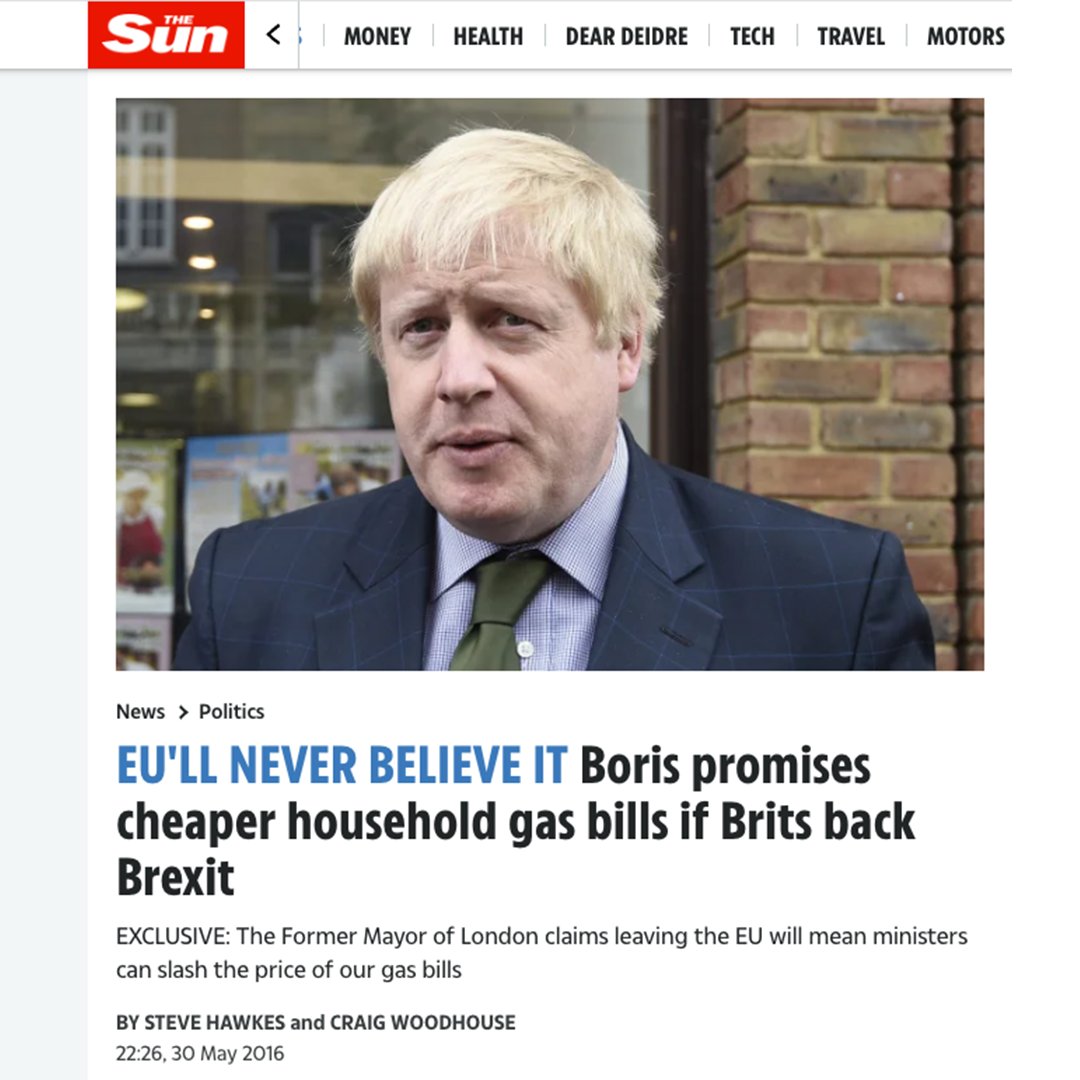This is a detailed desktop screenshot of The Sun's website, featuring a prominent news headline. At the top of the page, a navigation bar displays several options, though some are partially covered and may require scrolling to access fully. The visible options include Money, Health, Dear Deidre, Tech, Travel, and Motors.

The main headline centers around Boris Johnson, who is pictured posing in front of a business establishment with indistinct posters in the window behind him, and bricks visible to the left. The headline falls under the "News Politics" section and features a pun: "You'll Never Believe It." It reads, "Boris promises cheaper household gas bills if Brits back Brexit." The subheadline elaborates, "Exclusive: The former mayor of London claims leaving the European Union will mean ministers can slash the price of our gas bills."

The article is authored by Steve Hawkes and Craig Woodhouse, and it was posted at 22:26 on May 30, 2016.